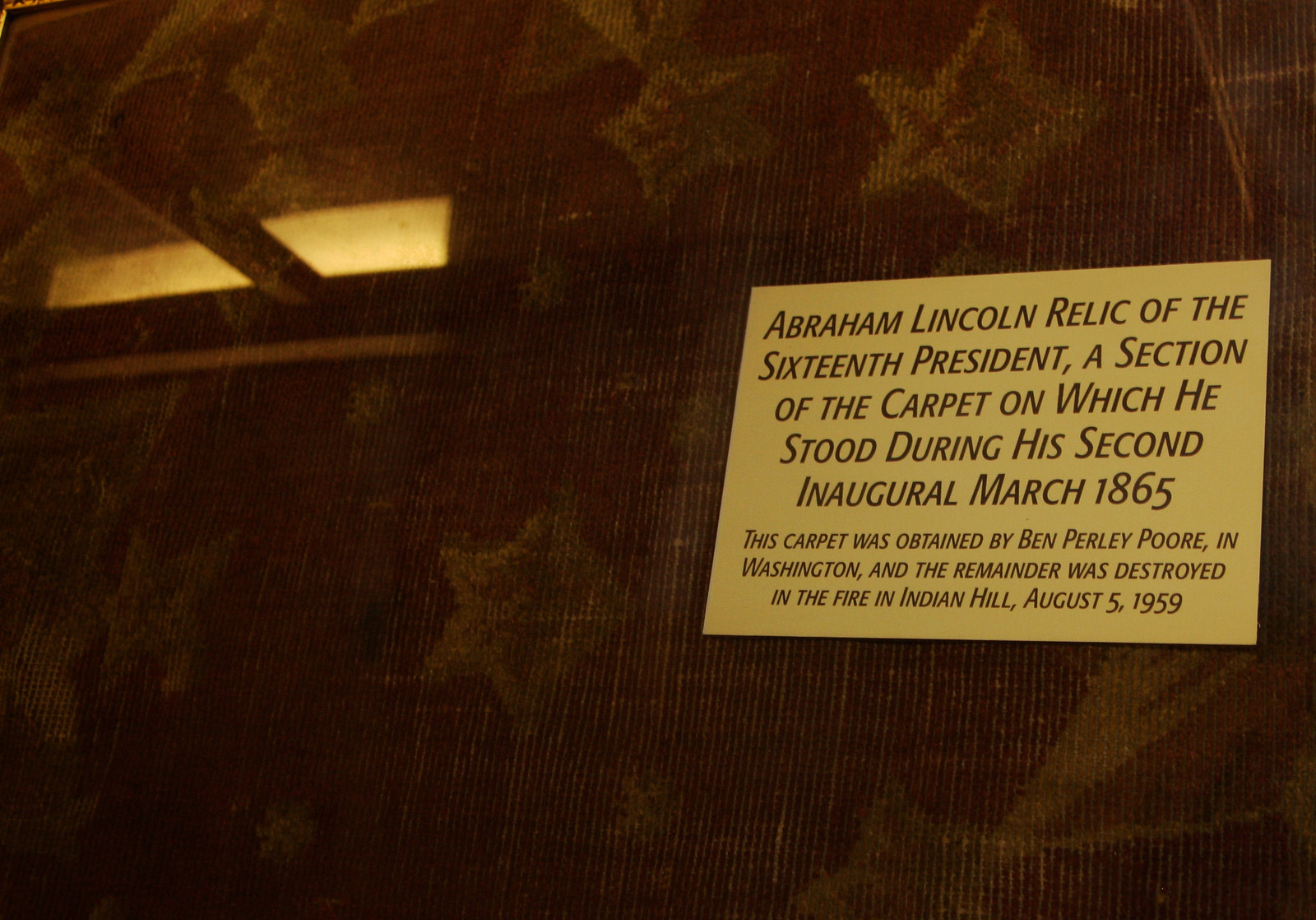The image is a horizontally oriented and very dark photograph with a brownish tone. A faint light emanates from the upper left corner, suggesting the presence of a window with partially closed shades. Dominating the background appears to be an old, rough carpet featuring a star pattern in red and yellow hues, seemingly hanging or displayed with care. On the right side of the image, there is a yellowish rectangular plaque with dark brown or black text. The plaque reads: "Abraham Lincoln, relic of the 16th President, a section of the carpet on which he stood during his second inaugural, March 1865." Below this prominent text, in a smaller font, additional information states that the carpet was acquired by Ben Pearlie Poor in Washington, and that the remainder of the carpet was destroyed in a fire at Indiana Hall on August 5th, 1959. This plaque appears to be applied either directly to the fabric or onto a picture frame or glass case surrounding the relic.